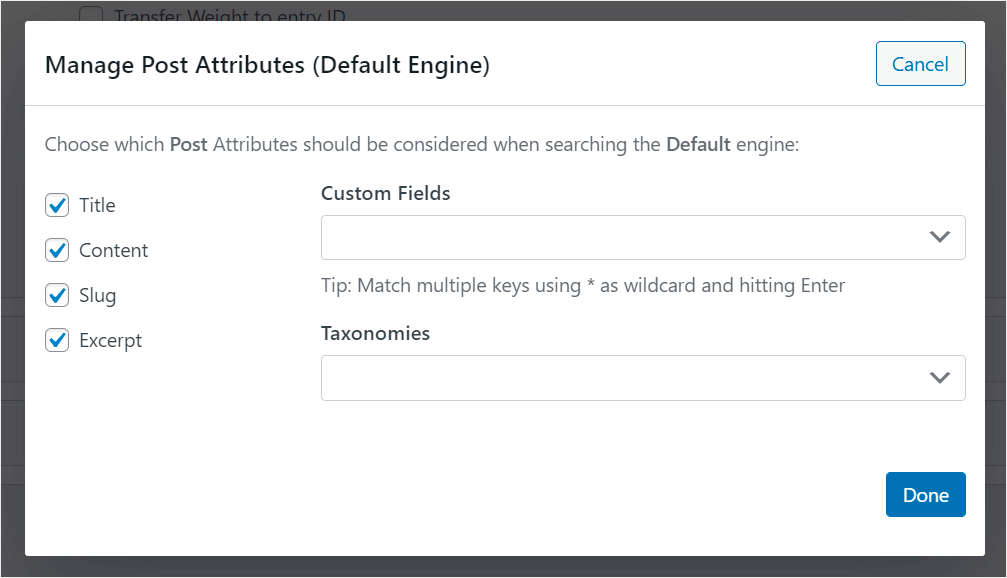This screenshot captures the "Manage Post Attributes (Default Engine)" settings window from a Windows computer, characterized by the distinctive dark blue interface typical of the operating system. The window is presented in a horizontal landscape format with a thick black border.

At the top, the title "Manage Post Attributes (Default Engine)" is bold and is followed by a horizontal separator line. Below the separator, a descriptive instruction reads, "Choose which post attributes should be considered when searching the default engine," with "Post" and "Default" in bold for emphasis.

On the left, a vertical column of checkboxes, all checked, lists the attributes: Title, Content, Slug, and Exit. To the right, two dropdown boxes are displayed. The first is labeled "Custom Fields," and adjacent to it is an elongated horizontal text box with a dropdown menu. Beneath this section, there's a tip explaining how to match multiple keys using the star (*) as a wildcard, accompanied by an actual star icon for clarity. 

Further down, the word "Taxonomies" precedes an additional dropdown box. In the bottom right corner, the “Done” button is prominent in blue with white text, while the “Cancel” button is positioned at the top right, styled with a white background, blue edging, and blue text.